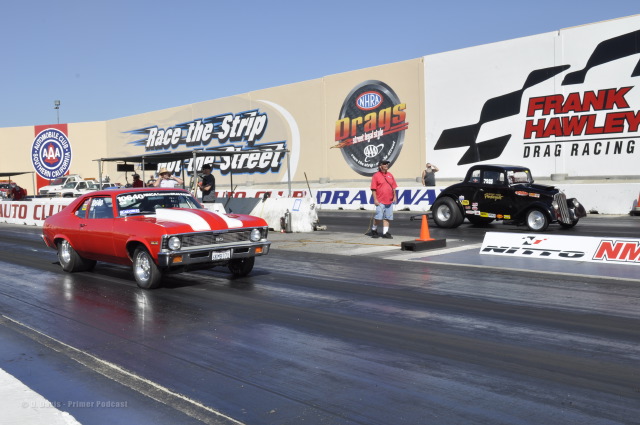The image depicts a drag racing event featuring a vibrant scene on a racetrack. At the forefront, prominently displayed on the left track, is a very old-looking red Mustang with distinctive yellow and white vertical stripes on the front of its engine hood, evoking a classic 1970s muscle car feel. To the right, on the second track, there's a small, black, dune buggy-like car which resembles an old-timey Model T from the 1930s. The background showcases a white wall adorned with various banners and sponsor logos. The wall has a striking black design, with "Frank Holley" in red text bordered in black, followed by another line reading "drag racing" in black text. Additionally, a tire-shaped logo with "NHRA" in white text above it and "drags" in orange is seen. Adjacent text in white states “race the strip,” likely part of the phrase "Race the Strip, Not the Street." In this dynamically detailed backdrop, there are also mentions of the Triple-A Automobile Club and Southern California, contributing to the vibrant, sponsor-rich atmosphere. Onlookers and participants populate the scene, including a man clad in a pink shirt and jean shorts standing near a pavilion, adding a human element to this energetic racing event.